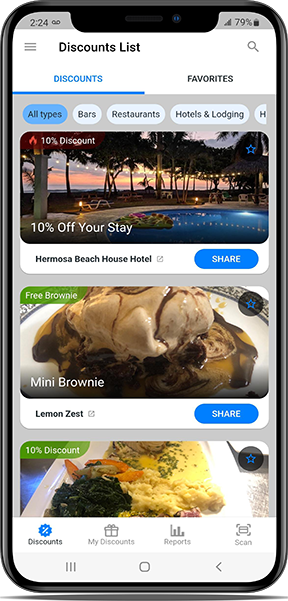In the image, there is a smartphone displaying a sleek, black-bordered touchscreen. At the top, the screen displays the time as 2:24, within a subtle gray bar. Directly below, a white header contains the text "Discounts list," flanked by a magnifying glass icon on the right and three horizontal lines on the left. Beneath this, highlighted in blue text, is the word "Discounts," and next to it, an unhighlighted "Favorites" tab.

Further down, there's a gray box showcasing an image of a tropical resort, likely a hotel, featuring a picturesque pool at sunset with trees adorned with string lights. Accompanying this image is the text "10% off your stay at Hermosa Beach House Hotel," followed by a blue "Share" button. 

The next section displays a green tag reading "Free brownie," with an image of a chocolate and ice cream-covered brownie on a plate labeled "Mini brownie," and underneath, "Lemon zest." Another blue "Share" button is present below this section.

Below, there is an image of a plate of food that appears to include shrimp, mashed potatoes, and spinach, with the caption "10% discount." 

The bottom part of the screen shows four icons labeled "Discounts," "My Discounts," "Reports," and "Scan." Beneath these icons, there are three vertical bars, a circular icon, and an arrow pointing to the left.